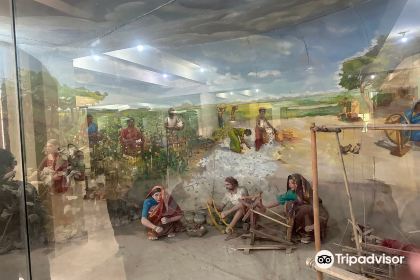This image is a low-resolution, slightly blurry photograph, seemingly sourced from TripAdvisor, depicting a museum exhibit behind a glass barrier. The exhibit features three lifelike mannequins arranged in a colonial-era setting. The figures are squat on the ground, engaging in traditional activities such as working with sticks and wood, possibly attempting to start a fire. The figure on the left appears to be a woman, donning a blue shirt and something over her head, with no shoes on. The backdrop includes a painted mural of an outdoor scene with greenery and wooden structures, evoking an ancient or farming period that may allude to the 1700s or Jesus' time. Lighting reflections and fixtures are visible on the glass, which slightly obscure the detailed view of the exhibit. In the lower right corner, the TripAdvisor logo, featuring a circular icon with an owl face in black and the text "TripAdvisor" in white, is present.